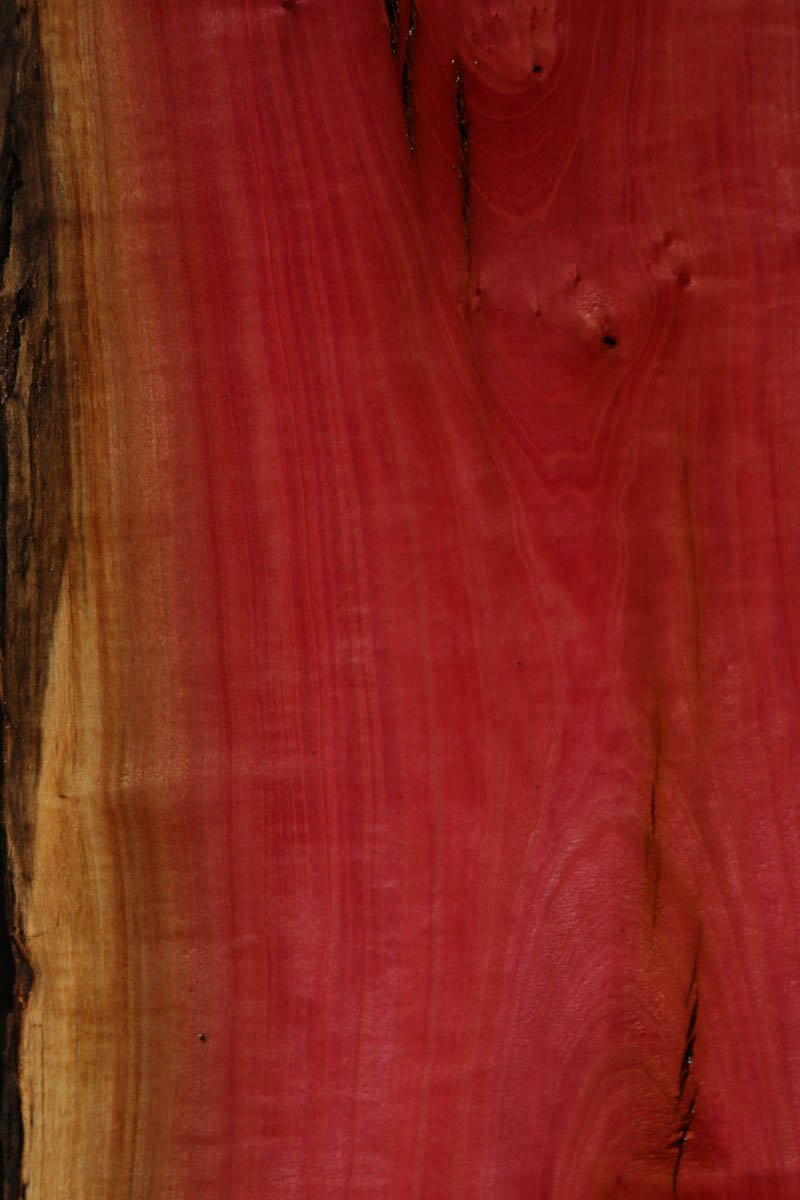The image showcases a close-up view of a freshly split piece of firewood. The wood, which seems to be artificially dyed or illuminated to appear an unnatural red, reveals a spectrum of colors. On the very left, the natural brownish-yellow hue of the wood is visible with darker brown lines marking the grain. Moving towards the center, the wood transitions through varying shades of brown to red, highlighting knots and intricate grains typical of cut firewood. Notable details include darker brown sections, small holes, and vertical cracks along the lower right, suggesting that the wood plank might be old or not well-maintained. The composition, bathed in what appears to be red lighting, captures the rustic texture and contrasts of the wood’s surface, illustrating a vividly detailed and freshly split piece of firewood.